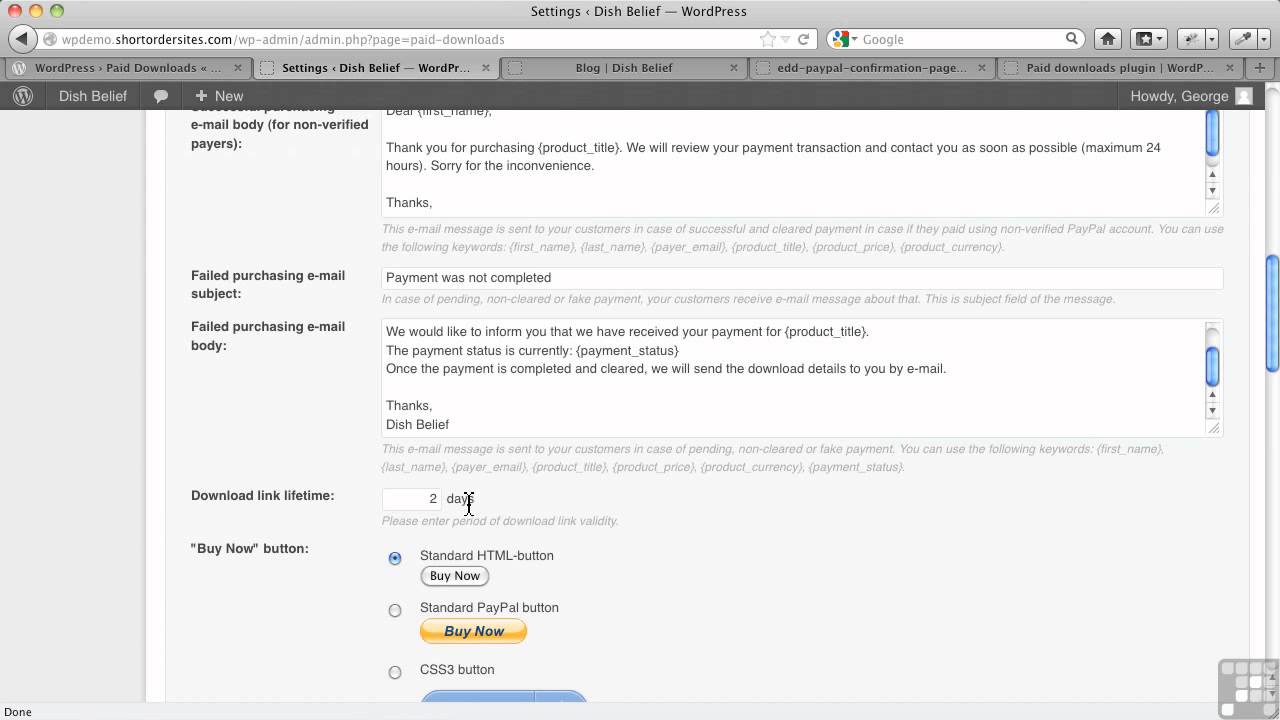The image displays a detailed view of the settings page for DishBeef-WordPress. On the left side of the screen, just outside a gray border, there are three colored buttons: a red circle, red button, yellow button, and green button. These likely represent window control buttons. Below these buttons is an address bar displaying the URL "citrus.com."

To the right of the address bar, there is a Google search box followed by several icons: a home icon, a star icon with a dropdown arrow, and two additional smaller icons that are unreadable. The current active browser tab is labeled "Settings-Dish." To its left is a tab named "WordPress-Paint" (though partially legible), and there are multiple other tabs to the right, which are unreadable.

Below the browser tabs is a black border that contains the WordPress icon and the text "Dash-Belief." To the right of this, icons for "Comment," "Plus New," and the word "New" can be seen. On the far right side, there is a greeting text "Howdy George" next to a user icon.

The primary content area of the settings page starts with a box titled "Email Body," which seems to be partially cut off, beginning with "Email body for non-verified players or payers." 

Further down, there is a section for "Failed purchasing email subject," containing the text "Payment was not completed." Below it, another box titled "Failed purchasing email body" includes a message notifying the user about their payment status with placeholders like "product_title" and "payment_status," ensuring that download details will be emailed once the payment is completed and cleared. The message ends with the signature "Thanks, Dash-Belief."

At the bottom of the page, there is a section labeled "Download link lifetime" specifying "two days." Below it, different types of "Buy Now" buttons are displayed, including a "Standard HTML button," a "Standard PayPal button," and a "CSS3 button." The "Standard HTML button" is shown as selected.